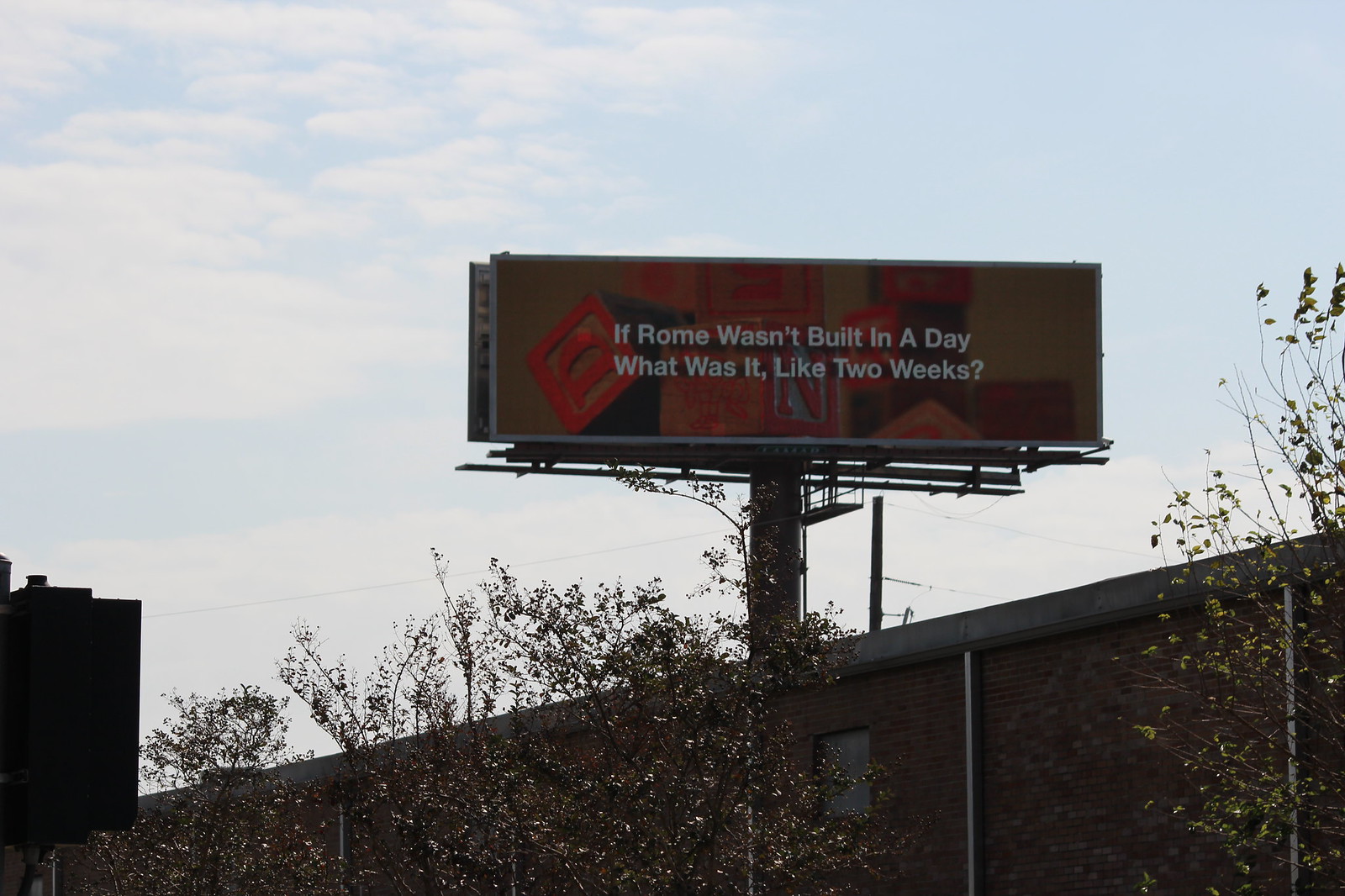The photograph captures an upward-looking perspective of a prominently positioned billboard against a predominantly blue, partly cloudy sky. The image is in landscape orientation, showing a building extending diagonally from the bottom left corner towards just below the midpoint on the right side. The sky, featuring scattered white clouds predominantly on the left half, forms the backdrop for the billboard. The billboard itself stands out with a humorous message in white text at the center, reading, "If Rome wasn’t built in a day, what was it? Like two weeks?" The billboard's background combines a browny-yellow hue with abstract red building block shapes, enhancing the overall visual appeal.